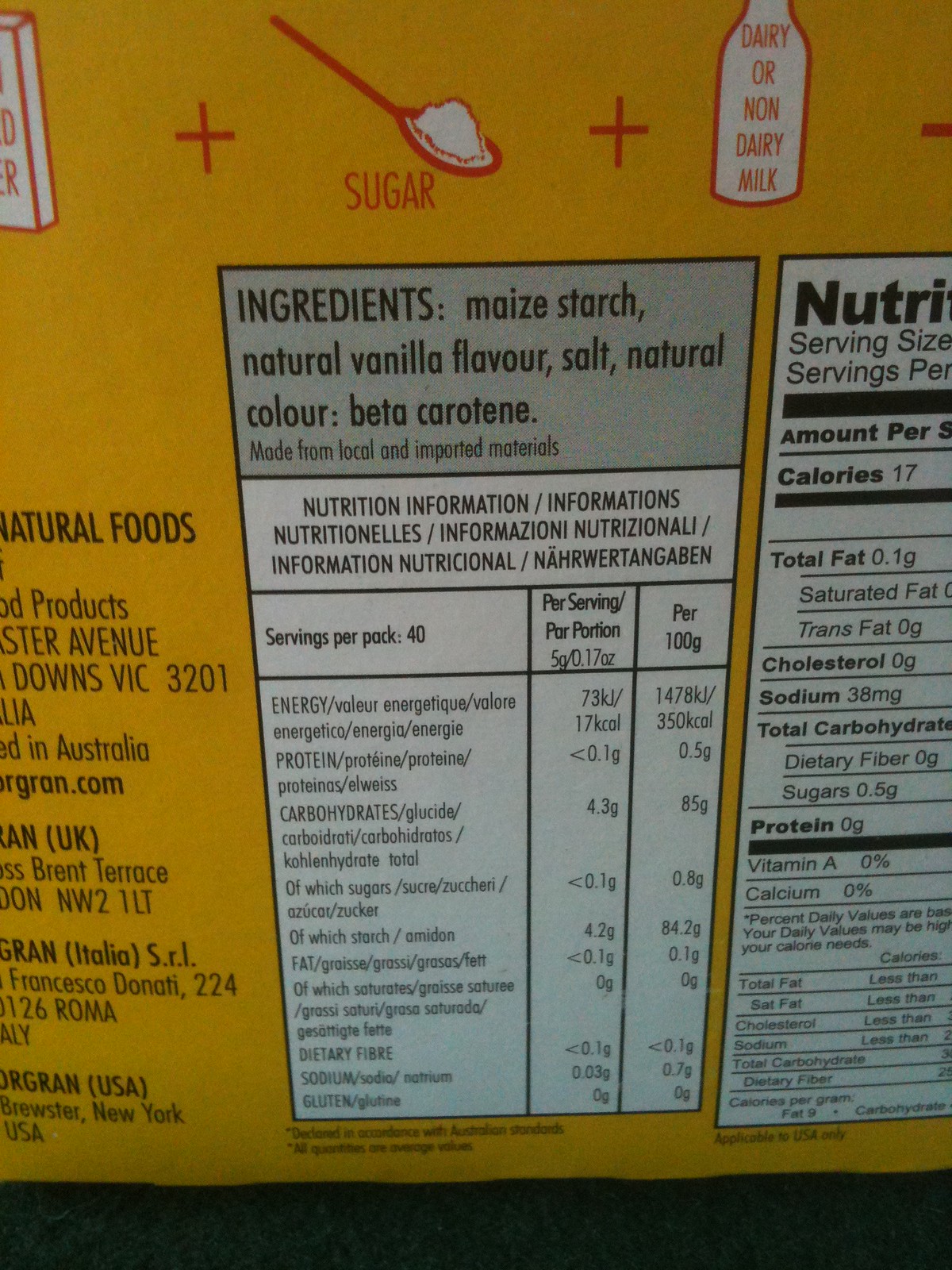This image showcases the label of a food or beverage product, prominently featuring a luxurious gold background. Central to the label, enclosed in a black border, is the ingredients list presented in gray text. Below this, within a white box, the nutritional breakdown is displayed for easy viewing. To the right, partially visible, is the nutrition facts panel beginning with the letters "NUTRI."

The ingredients listed include maize starch, natural vanilla flavor, salt, and natural color (beta carotene). Notably, the product offers 40 servings per pack. The nutrition facts panel reveals critical nutritional information per serving: 17 calories, 0.1 grams of total fat, 38 milligrams of sodium, 0.5 grams of sugars, and 0 grams of protein.